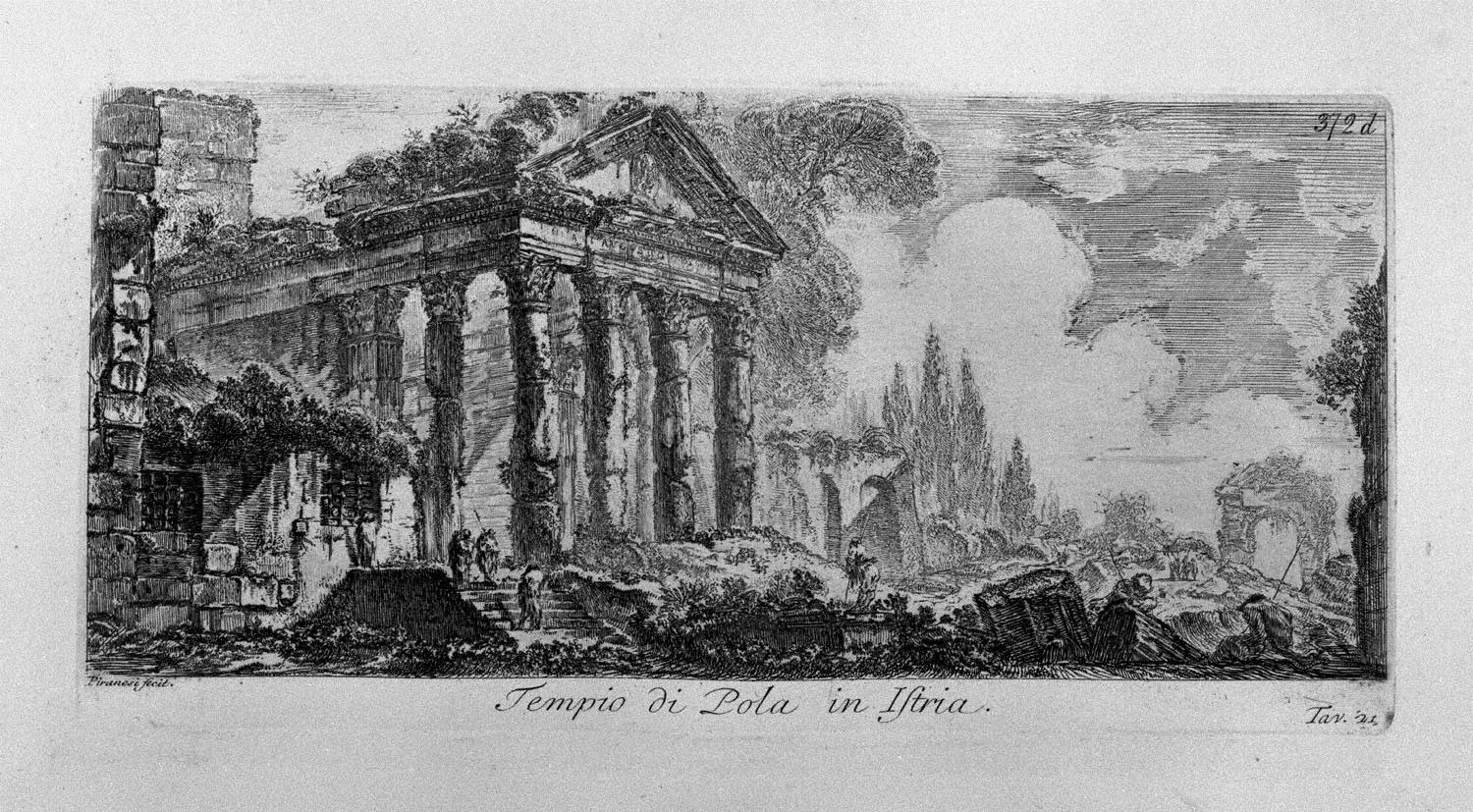This monochromatic scan portrays a detailed pen and ink drawing of ancient ruins, possibly of Roman origin, embodying classical architectural elements. Central to the image is an imposing structure resembling a temple or cathedral entrance, marked by a triangular pediment supported by four prominent columns, with additional columns extending into the background. The structure appears aged and partially deteriorated, with sections of the roof crumbling and debris scattered around its base. On the left, a stairway ascends towards the building, populated by several figures walking up and down. On the right side of the structure, trees and clouds add depth to the scene. Specific text annotations include "372D" in the upper right, "TAV 21" in the lower right, and the Latin phrase "Tempio di Pola in Ifria" at the bottom, hinting at its historical or geographical significance. Overall, the artwork captures the grandeur and decay of classical ruins amidst a serene landscape.